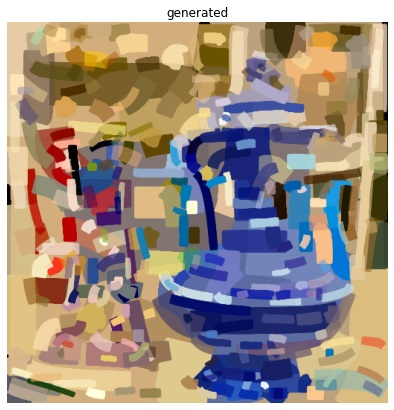The image is pixelated and not clearly visible, with a mix of colors making up the scene. At the top of the image, black text reads "generated." The central focus appears to be a painting or drawing featuring an object resembling a vase or trophy with handles on both sides. This object is predominantly composed of shades of blue—both light and dark—and interspersed with white accents. Surrounding the object is a background predominantly filled with brown and dark brown hues, though black is also present in various parts.

On the left side of the image, there’s another object whose details are unclear. This secondary object is painted in a variety of colors including brown, pink, purple, orange, blue, dark blue, dark green, red, and light red. The background, continuing to be variegated, includes brown, dark brown, green (particularly in the top left), gray, and dark purple shades, merging into an eclectic mix of colors. This complexity in colors adds a layer of abstract artistry to the overall composition, despite its pixelation and lack of clear visibility.